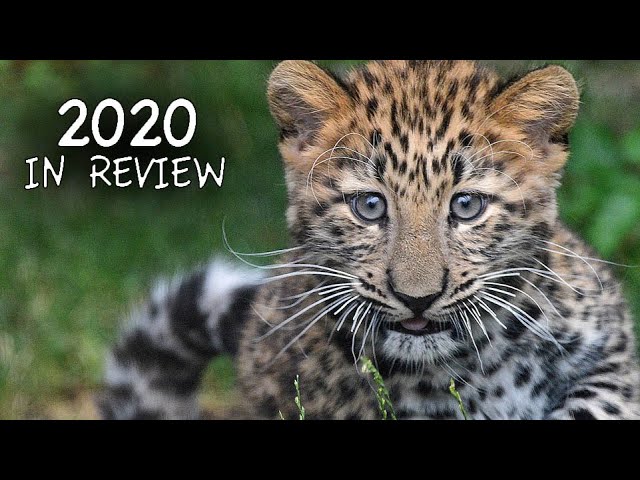The photo features a captivating young cub, possibly a leopard or cheetah, looking directly at the camera with strikingly inquisitive eyes. The cub's fur is a beautiful blend of brown and tan hues, accentuated with black spots throughout and complemented by prominent white patches on its belly and whiskers. Its long white whiskers and slightly protruding pink tongue add to its endearing appearance. In the backdrop, which is slightly out of focus, lush green vegetation provides a natural setting for the cub. The image is framed with black borders on the top and bottom, resembling an old TV screen format. In the top left corner, white text reads "2020 in review," suggesting the photo might be part of a retrospective collection or slideshow.